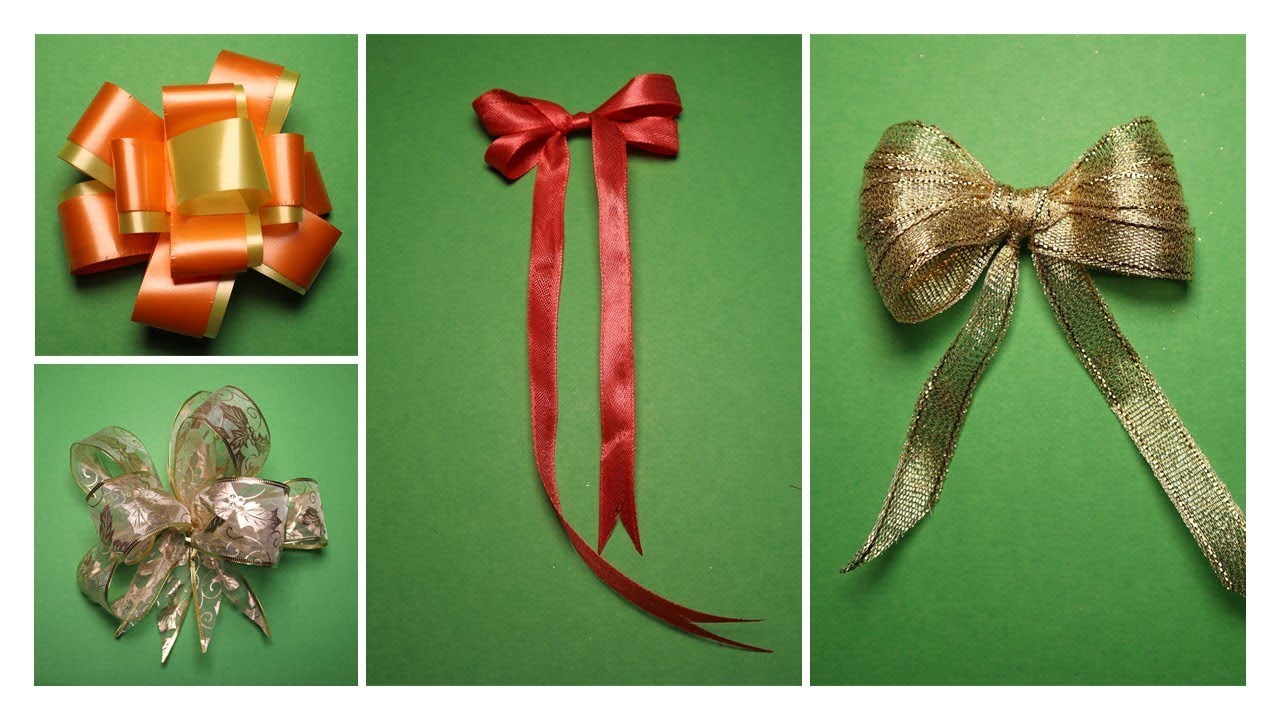This image is a collage of four photographs displaying various decorative bows set against a solid green background, separated by thin white lines. In the upper left, there's an elaborate bow made from many folded pieces of orange and yellow (or gold) ribbon, forming a starburst or flower pattern. Directly below it, a bow constructed from a thin, almost lacy, silver material features areas of transparency and gold leaf design, creating an intricate, folded effect.

In the center, a classic-style bow made from glossy red fabric is showcased. This bow, which resembles a shoe knot, has two long tails that extend downward. Lastly, on the right, the image presents a closer view of a gold mesh fabric bow, crafted in a simple style with two short tails angled downward, forming an 'A' shape.